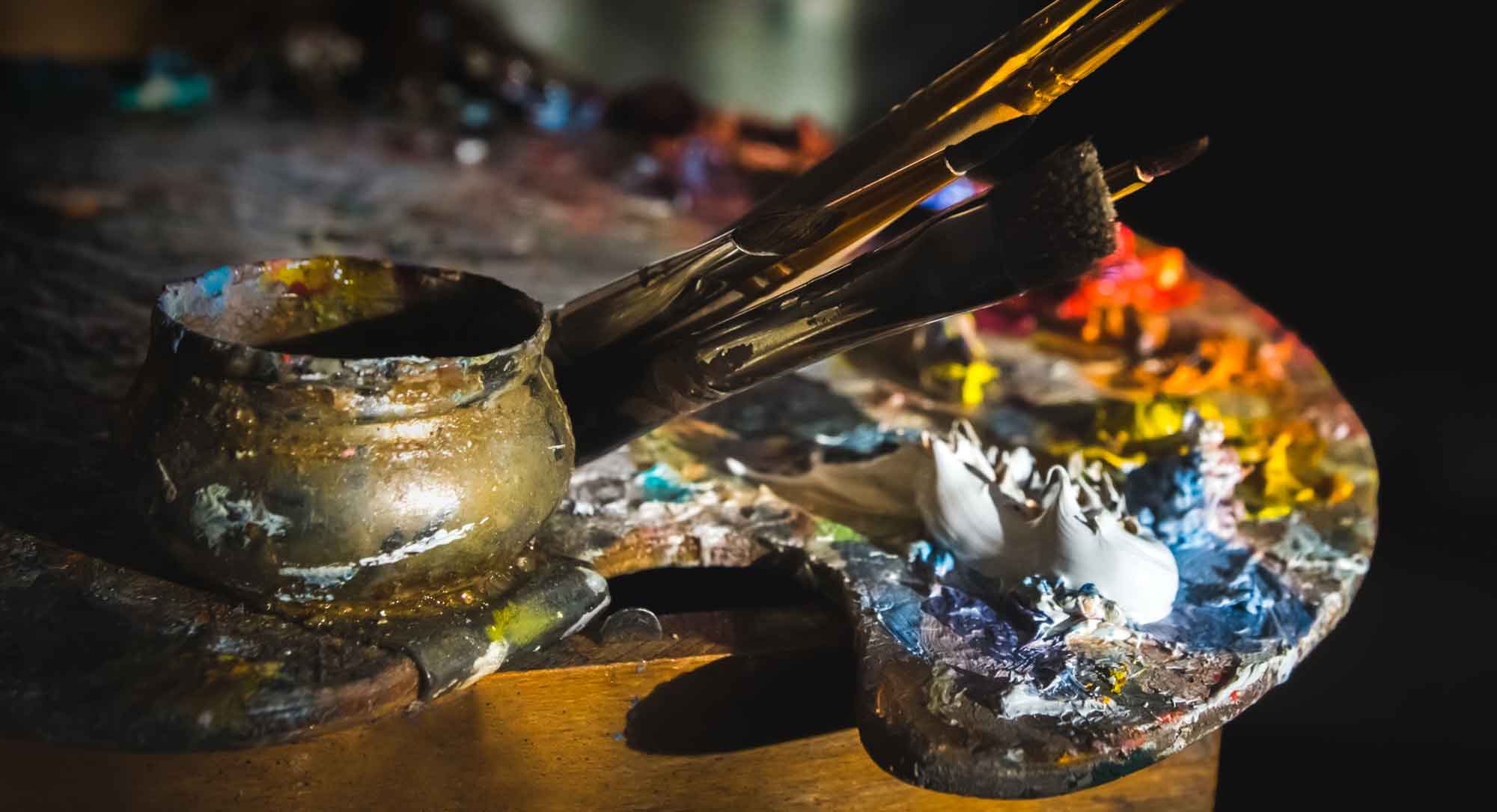An up-close photograph showcases a heavily-used oval-shaped wooden artist’s palette. The background is pitch black, with some bright lighting striking from the right side, highlighting the detailed textures and colors of the palette. The palette rests on an old wooden surface, perhaps a table or chair. On the left side, there's a small, metallic bowl, likely copper or bronze, serving as a rinse cup for paint or water. The palette itself is cluttered with a plethora of colorful paints, prominently featuring a glob of white paint in the foreground, with bright splashes of blue, yellow, orange, and red, along with smeared and mixed colors across its surface. Nestled against the bowl, a collection of six or seven paintbrushes of various sizes jut out, pointing towards the upper right. The palette gives an impression of a well-loved and frequently used artist’s tool, with paint clumps and smears indicating its continuous use without frequent cleaning.